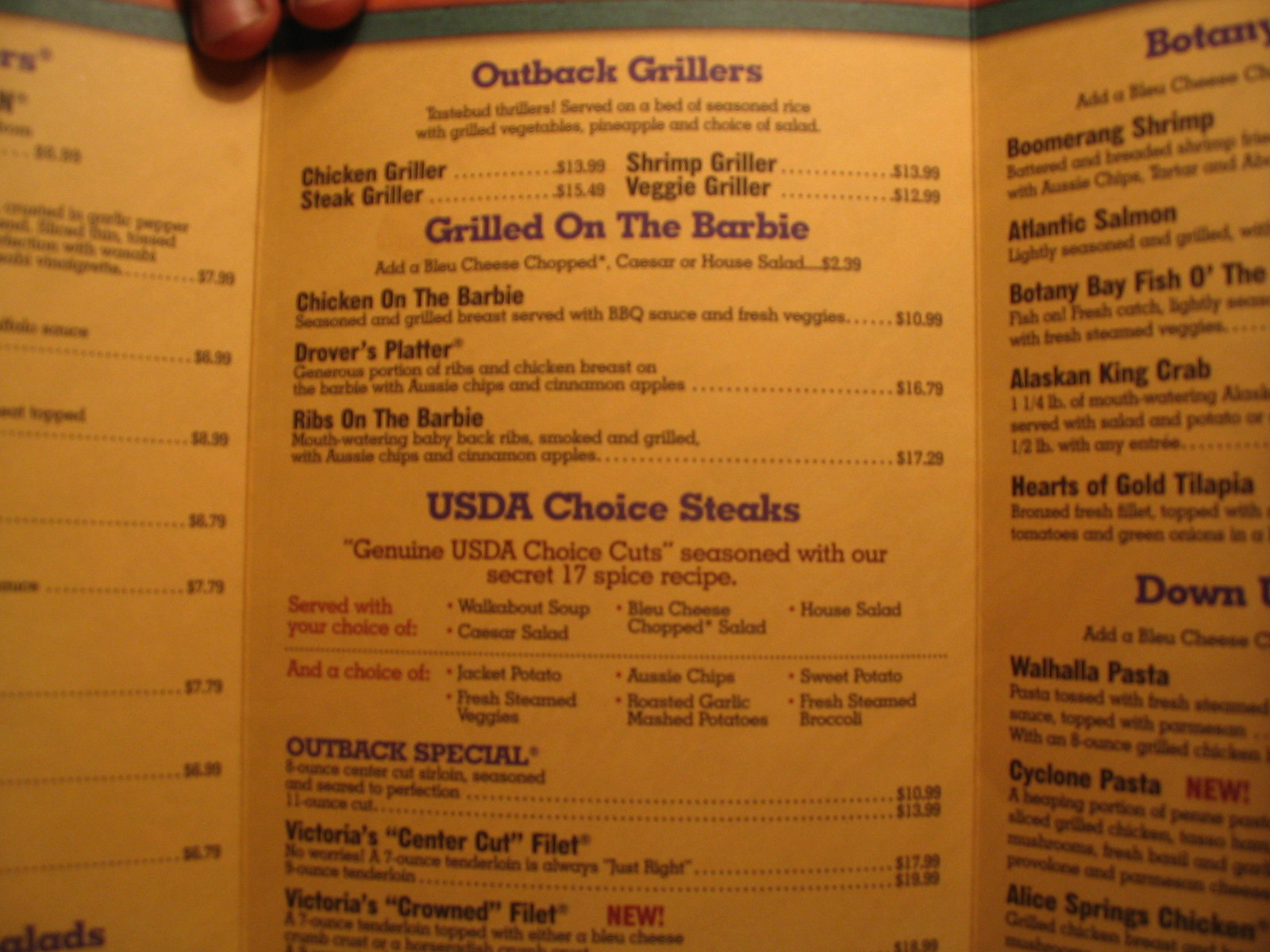The image captures a photograph of a three-panel, beige-colored paper menu, held up by two dark fingers visible in the upper left corner. The text on the menu is predominantly black with occasional red highlights. The central panel prominently features the heading "Outback Grillers," listing items such as Chicken Griller ($13.99), Steak Griller ($15.49), Shrimp Griller ($13.99), and Veggie Griller ($12.99), all served on a bed of seasoned rice with grilled vegetables, pineapple, and a choice of salad. Below this, there's a section titled "Grilled on the Barbie" with options like Chicken on the Barbie ($10.99), featuring a seasoned and grilled breast served with barbeque sauce and fresh veggies. Also listed is the Drover's Platter ($16.79), with ribs and chicken breast served with Aussie chips and cinnamon apples, and Ribs on the Barbie ($17.29), described as mouthwatering baby back ribs smoked and grilled, also served with Aussie chips and cinnamon apples. On the right panel, under headings like "USDA Choice Steaks" with options such as Outback Special and Victoria's Center Cut Filet, there's a variety of dishes including "Boomerang Shrimp," "Atlantic Salmon," "Botany Bay Fish-O-the-Day," "Alaskan King Crab," "Hearts of Gold," "Tilapia," "Walhalla Pasta," and "Cyclone Pasta," along with "Alice Springs Chicken." Despite some cut-off portions and difficult-to-read areas, the menu clearly represents a detailed listing of offerings from what appears to be an Outback Steakhouse.